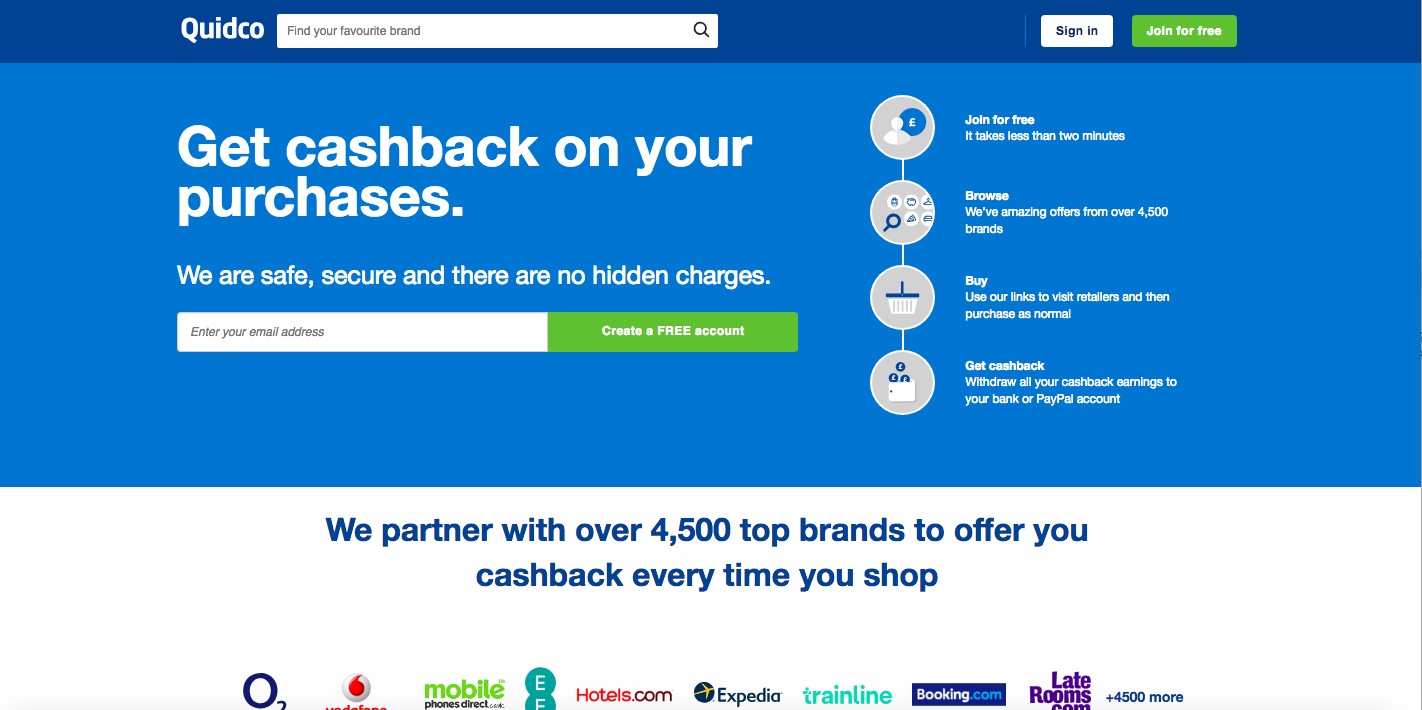This is an image of the Quidco website homepage, featuring a prominent dark blue header bar. The header includes the Quidco logo in white font on the left, a search bar with the placeholder text "Find your favorite brand," a white "Sign In" button in black font, and a green "Join for Free" button with white font.

Beneath the header, a large white text reads "Get cash back on your purchases." Below this, in smaller white font, a reassuring message states, "We are safe, secure and there are no hidden charges." Underneath this message, there's a white input field for entering an email address, accompanied by a green "Create a Free Account" button.

Further down, a vertical series of four circular icons describe the process of earning cash back with Quidco. The first icon depicts a person with a small blue circle behind the head, and the caption reads, "Join for free. It takes less than two minutes." The second icon shows a magnifying glass over some icons, alongside the text, "Browse amazing offers from over 4,500 brands." The third icon features a bag or shopping cart, with the text reading, "Buy. Use our links to visit retailers and then purchase as normal." The fourth icon depicts coins falling into a wallet, with the caption stating, "Get cash back. Withdraw all your cash back earnings to your bank or PayPal account."

The section below this blue area transitions to a white background with dark blue font, announcing, "We partner with over 4,500 top brands to offer you cash back every time you shop." At the bottom of the page, logos of various partner companies are displayed, including Mobile Phones Direct, Hotels.com, Expedia, Trainline, Booking.com, and Laterooms.com, among others. The text mentions there are 4,500 more brands available, with some logos being too small to read clearly.